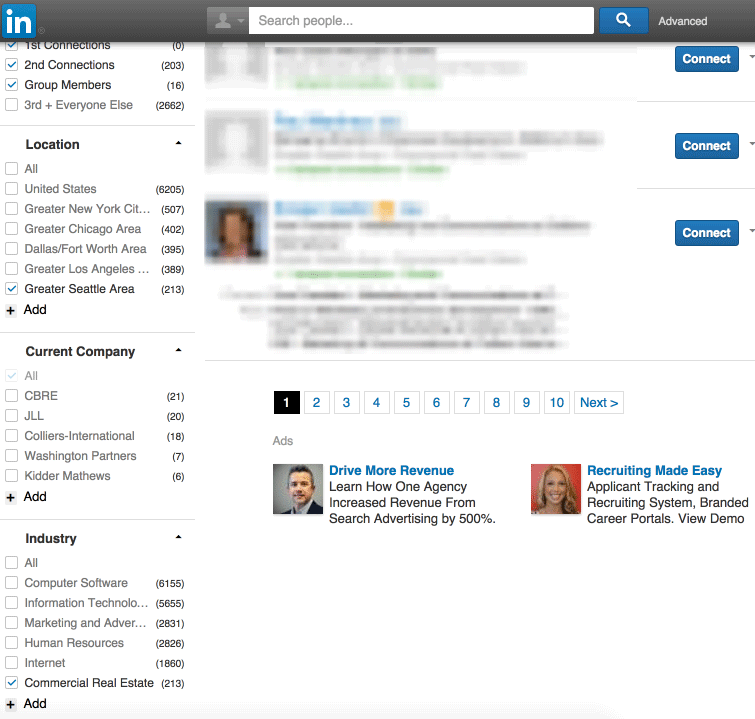This screenshot from LinkedIn showcases its user interface and search options. In the top left corner, a blue square with the white letters "IN" marks the LinkedIn logo against a dark grey toolbar that spans the width of the screen. Centrally located at the top is a search bar labeled "Search people," accompanied by a blue search button with a white magnifying glass, and an "Advanced Search" option to its right.

Below the toolbar, three profile cards are visible, each obscured for privacy, all prominently featuring blue "Connect" buttons to their right. A navigational bar beneath these profiles lists page numbers 1 through 10, with the first page selected in black. 

Further down, two advertisements are displayed. The first ad features a square image of a Caucasian man in a grey shirt and black or dark grey suit jacket against a grey background, promoting a search advertising success story with the headline, "Drive more revenue—Learn how one agency increased revenue from search advertising by 500 percent."

Adjacent to this, a second ad includes an image of a smiling Caucasian woman with long blonde hair set against a burnt orange background. The text promotes recruiting solutions with the tagline, "Recruiting made easy—Applicant tracking and recruiting system, branded career portals, view demo."

On the far left of the screenshot are filtering options for refining profile searches by criteria such as current company and industry.